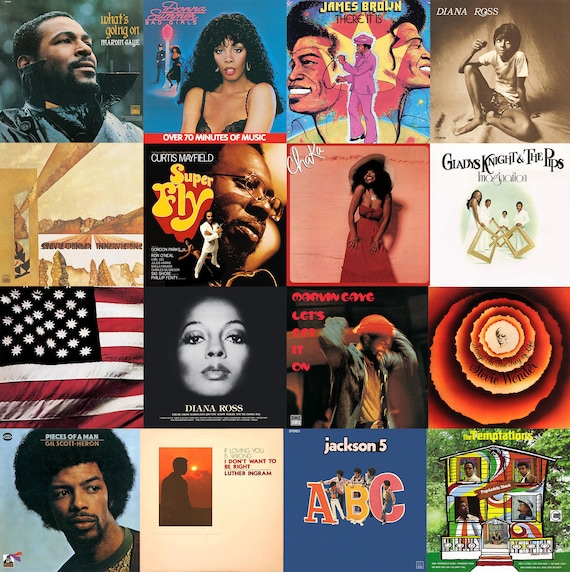The image is a vibrant square collage of 16 album covers, predominantly featuring iconic R&B and Motown artists from the 70s and 80s. The top-left corner showcases Marvin Gaye's "What's Going On," followed by Donna Summer's disco album "Bad Girls," and James Brown's "There It Is." Diana Ross appears twice, one cover showing her in black and white, sitting on the ground. Curtis Mayfield's "Superfly" and Gladys Knight & the Pips, with the group holding empty frames against a mostly white background, are also included. The collage features a kaleidoscope of colors, capturing the rich diversity of album art from this musical era. Other notable albums include the Jackson 5's "ABC," Stevie Wonder, Chaka Khan in a red dress, a patriotic album cover with a distinctive American flag, Luther Ingram's "If Loving You Is Wrong, I Don't Want To Be Right," Jill Scott, and Gil Scott-Heron's "Pieces of a Man." The top-down view allows for an appreciation of all the album covers simultaneously.